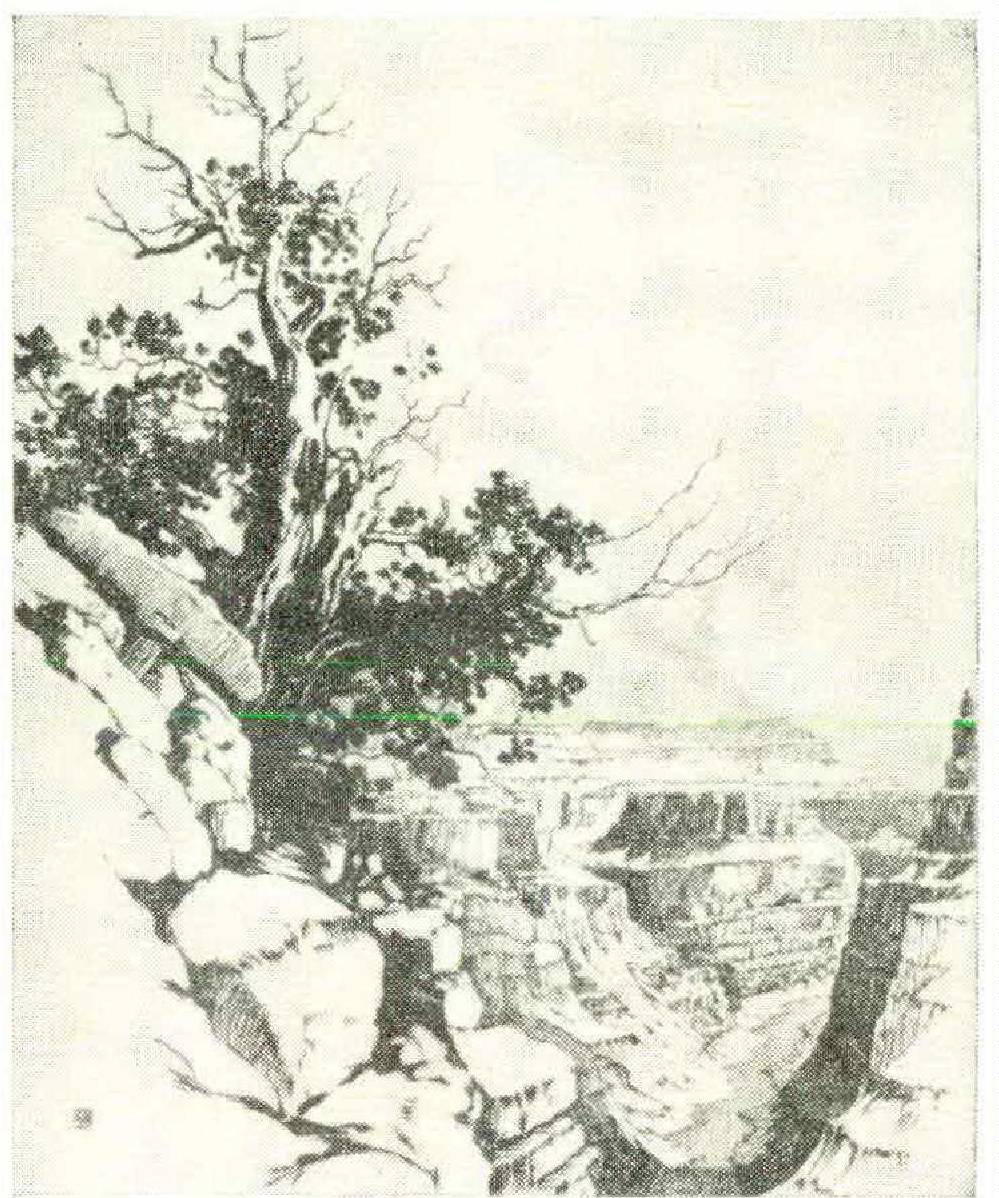This image portrays a vintage, black-and-white sketch of the Grand Canyon, exuding an antiquated charm. The scene is illustrated through cross-hatching or a similar technique, contributing minor shading details. The aged quality is highlighted by yellowed nuances, and green streaks suggest it might be a scanned copy with printer artifacts. A prominent feature in the foreground is a ragged tree on the left side, partly bare with sparse leaves mainly on its lower branches, rooted in a rocky mound. In contrast, the right side reveals a vast canyon with silhouettes of broken and large rocks descending into the depths. Far in the distance, flat-topped plateaus amplify the expanse of this rugged landscape.